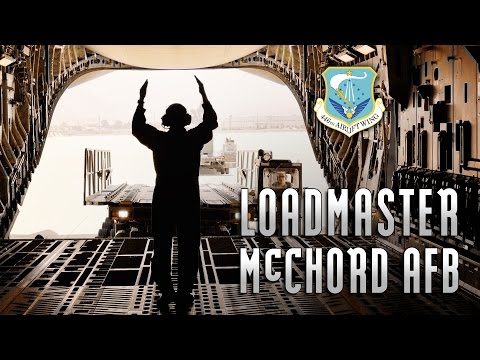The image is an advertisement likely associated with an Air Force base. It prominently features a silhouetted person, possibly an air traffic controller or loadmaster, raising their arms as if directing air traffic or coordinating the loading of equipment. The individual is equipped with a headset and stands within a structure that appears to be a hangar bay, possibly connecting machinery or aircraft ramp to a hangar door. The backdrop reveals a faint skyline, adding depth to the scene.

In the upper right corner of the image, there’s a military-related emblem with a ribbon at the bottom. The emblem likely represents the 446th Airlift Wing with its blue and white design featuring a bird and other intricate details. Dominating the lower right corner of the image, the text "LOADMASTER MCCHORD AFB" is boldly displayed in white and silver, with "MCCHORD AFB" presumed to stand for McChord Air Force Base. The overall color palette of the image includes dark brown tones, balanced by the striking white text and emblem details.